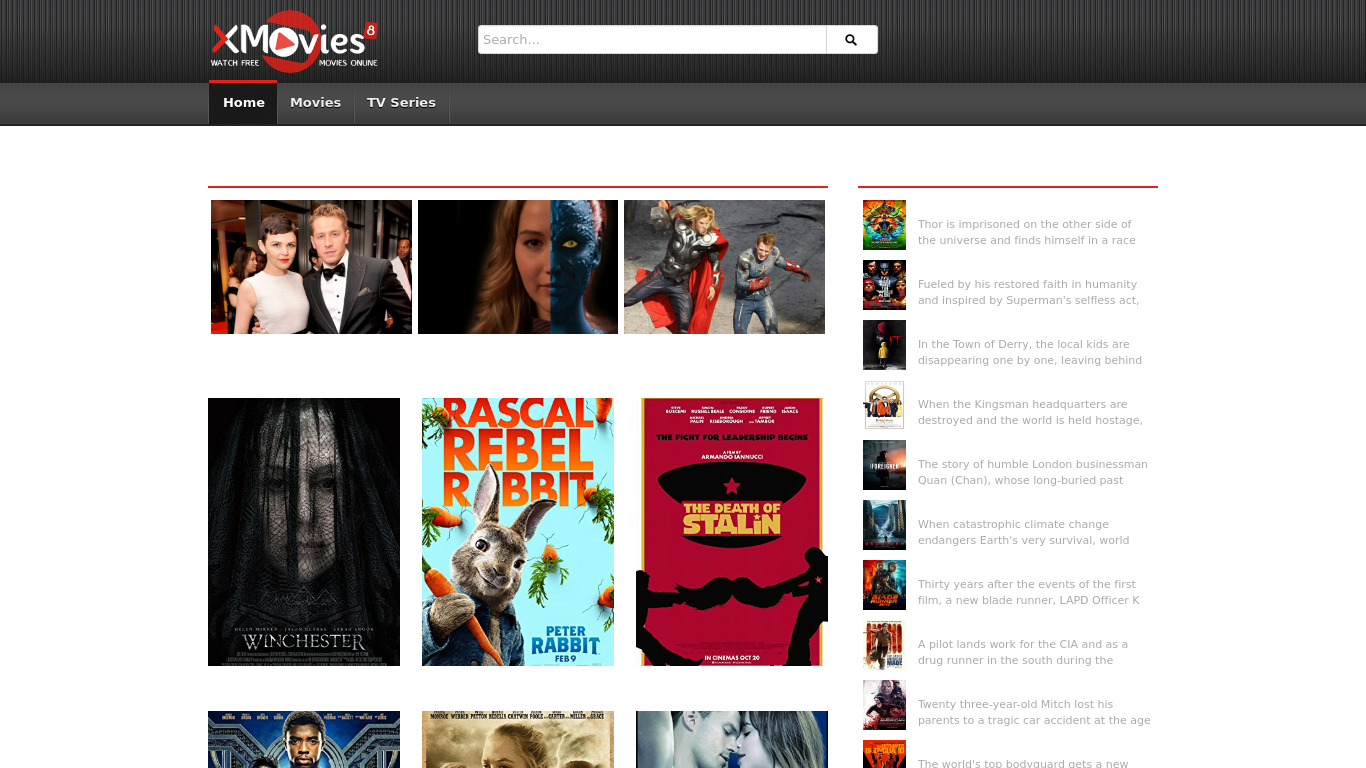The image appears to be a screenshot from a streaming platform named "X Movies." The "X Movies" logo features an "O" with a play button in the middle, set against a red circle. Below the logo, there's the tagline "Watch for your movies online," and on either side of the logo, there are search fields, one being located to the right.

The navigation menu below includes options for "Home," "Movies," and "TV Series," with "Home" currently highlighted, indicating the user is on the home page.

Displayed prominently are three images. The first image depicts a red carpet event with elegantly dressed attendees. One person is wearing a suit and bow tie, while a woman in a white dress stands next to him. Among the celebrities present are the actress who plays Mystique in the X-Men movies and another actress known for her role in "The Hunger Games." Additionally, Chris Hemsworth, known for his roles in various movies including playing Thor, is also visible.

Below these images, there are larger movie cover art images. Titles include "Winchester," a horror film; "Peter Rabbit," a family movie; "The Death of Stalin," a historical satire, and partially visible are covers for "Black Panther" and two other films cut off from the view.

To the right of the main section, there's a column featuring several articles with thumbnails. Headlines include "Thor is in prison on the other side of the universe" and "Restored faith in humanity inspired by Superman's selfless act." These smaller box art images and accompanying snippets are designed to entice viewers into watching these movies.

Overall, the screenshot captures a well-organized, vibrant homepage filled with high-quality images and enticing headlines designed to attract viewers to various films and articles.